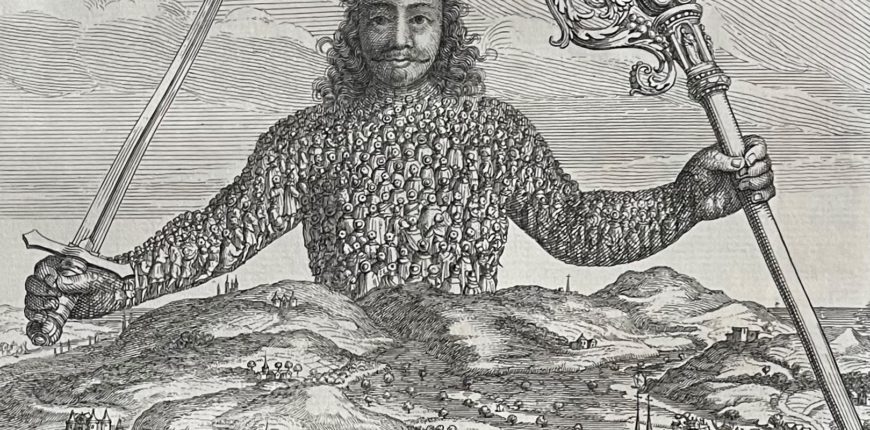The detailed black-and-white line drawing depicts a close-up image of a person visible from the waist up, embodying a stylized, almost mythical figure. The person, adorned with long curly hair, a handlebar mustache, and a goatee, holds a sword in their right hand pointed diagonally upwards and a staff or pole in their left hand angled downwards. Intriguingly, the person’s body is composed of numerous tiny images of other people, woven together to form the whole. In front of this figure lies a serene farming landscape with rolling hills, a handful of trees, and sparse buildings, stretching out towards the right where water can be seen in the background. The entire scene, reminiscent of an old woodblock print, is filled with detailed, wavy lines, adding to its ancient and intricate appearance.